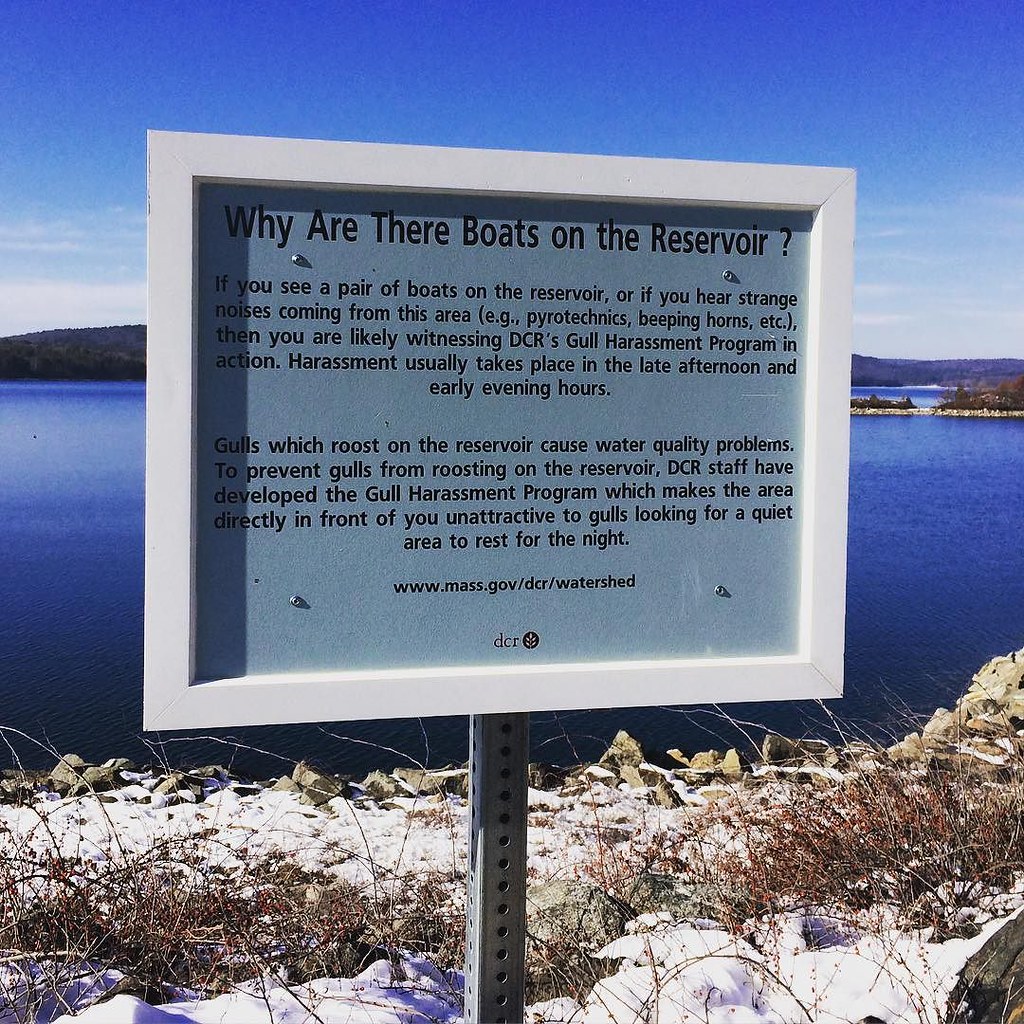In the image, there is an informational sign next to a large reservoir, prominently surrounded by a vibrant bright blue sky with wispy clouds framing either side of the sign. The background scenery features a gently rising hill partially covered in vegetation, with the hues of the deep blue water blending into lighter blue shades. On the right-hand side, a small piece of land juts into the water, dotted with shrubs and bushes. The bank, where the sign is situated, is rocky and covered in snow with scattered shrubbery and twigs.

The sign is mounted on a metal pole with holes, framed in white wood with a silver inner panel. It prominently reads in black text: "Why are there boats on the reservoir?" The sign explains the DCR's gull harassment program, which is meant to deter gulls from roosting on the reservoir to prevent water quality issues. The program usually takes place in the late afternoon or early evening and employs methods like pyrotechnics and beeping horns to make the area unattractive to gulls. The sign includes the website www.mass.gov/DCR/watershed along with a DCR logo featuring a flower at the bottom.